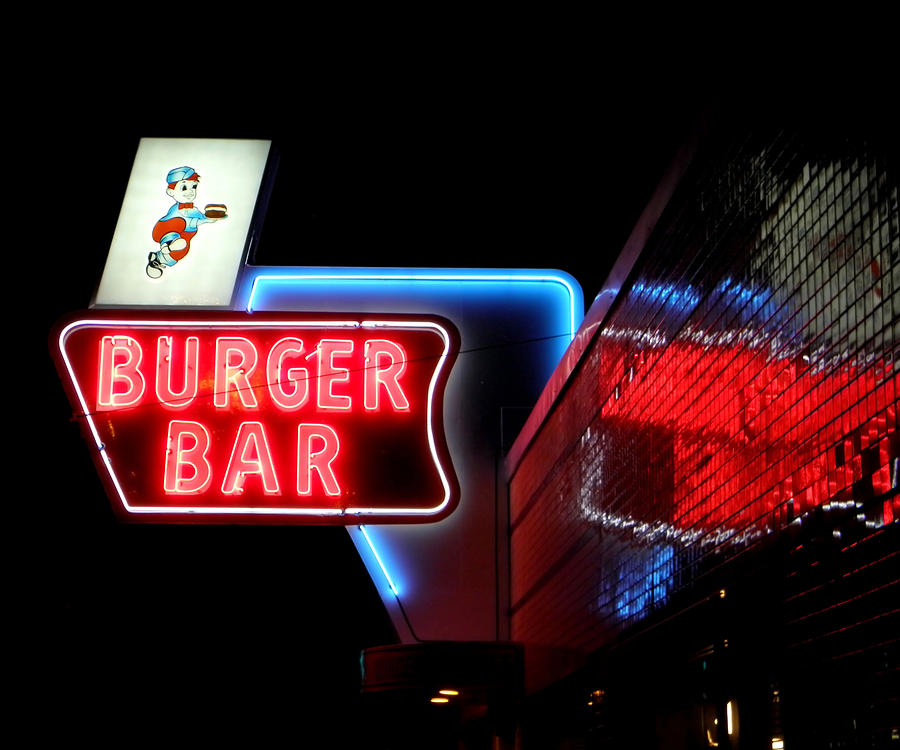This photo captures a vibrant neon sign prominently displayed atop a building at night. The sign reads "Burger Bar" in bold, red neon letters outlined in white, glowing brightly against the dark background. Above the text, there is a whimsical illustration of a boy with red hair, donned in a blue cap, blue shirt, and red pants, holding a burger. The boy is depicted standing on one leg, possibly in a running pose, ready to deliver the burger. The sign is supported by a blue neon pillar that also adds to the overall illumination. The building’s front features reflective, mirror-like tiles that echo the vivid colors of the neon lights. Additional indirect lighting is seen underneath the roof overhang, enhancing the visibility of the sign against the night sky. The entire scene is bathed in the vibrant glow of the neon, making the sign the focal point amidst the dark surroundings.